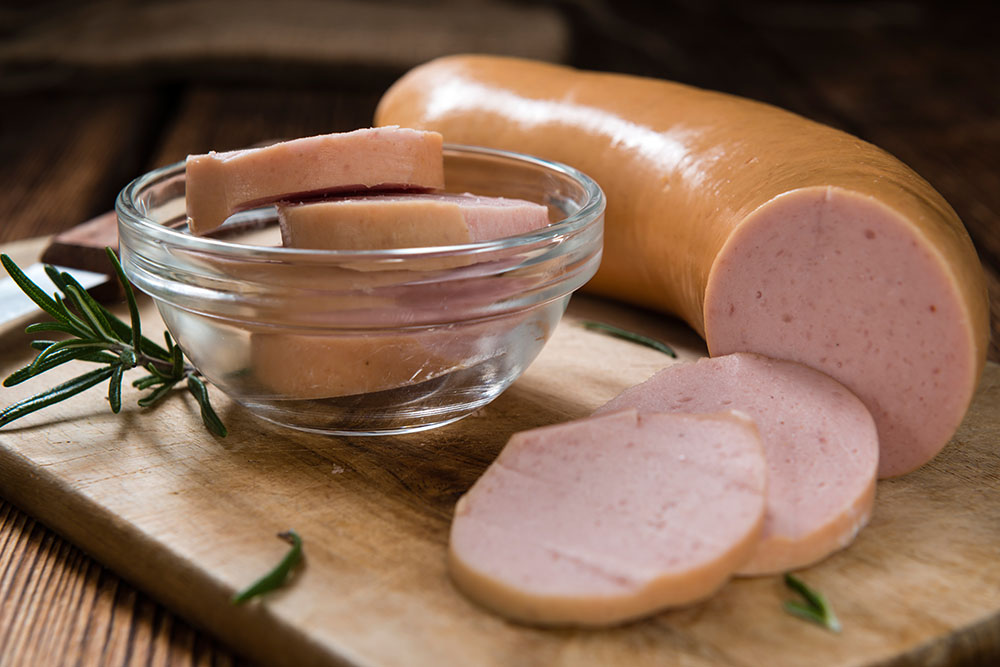In the carefully staged photograph, a wooden cutting board of high quality and warm brown color rests atop a wooden table. Centered on the cutting board is a large, tubular piece of meat, resembling a strip of bologna or sausage, partially sliced into thin, quarter-inch pieces. Two of these slices are meticulously placed directly in front of the larger, uncut section. The remaining slices, approximately three to four in total, are organized in a small, clear glass bowl positioned to the left of the larger meat piece. Adjacent to this arrangement, a few sprigs of green leaves, possibly evergreen, lie artfully, with some individual leaves scattered around for decorative effect. In the background, the wooden handle and the metal blade of the cutting knife can be discerned, adding to the rustic culinary aesthetic.